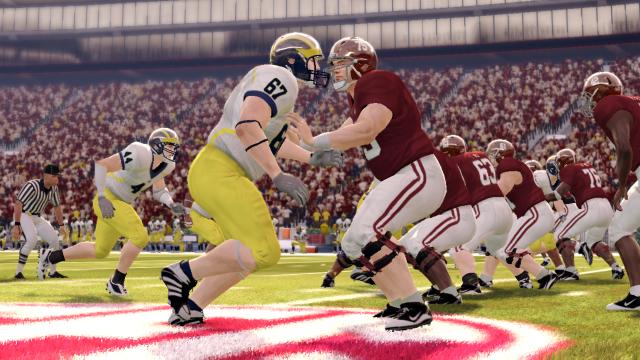In this zoomed-in gameplay screenshot from a football game, the image captures a tense moment likely from a college match, as deduced by the team colors which do not match typical NFL palettes. The players are seen in action on the field, with the offensive team clothed in red and white uniforms preparing to execute a pass. On the right side of the image, the defensive team, dressed in yellow, blue, and white, is aggressively rushing towards the quarterback. The stands in the background are filled with enthusiastic fans, primarily wearing white and red, which adds to the collegiate atmosphere of the scene. The focus is on a player on the left-hand side who appears to be bracing himself to fend off the incoming defense, highlighting the intensity and strategic maneuvers characteristic of football gameplay.